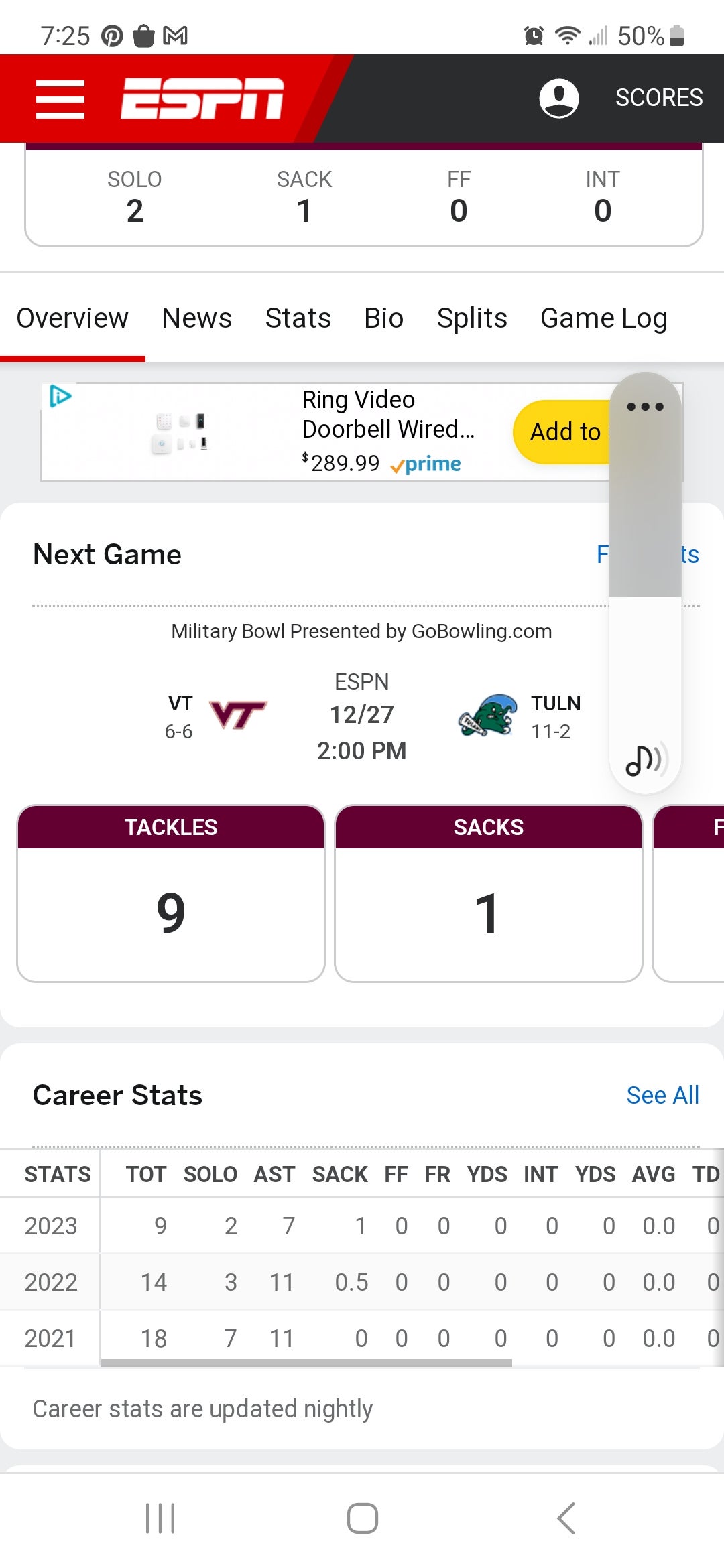In this image, set against a clean, white background, there is a screenshot of a mobile application interface. In the upper left corner, with a white backdrop, the time is displayed as '7:25' in crisp black text. Just to the right of the time, icons for a shopping bag and Google Mail are visible, suggesting notifications or shortcuts.

In the upper right corner, the Wi-Fi icon is lit but only shows one bar out of five, indicating a weak connection. Next to the Wi-Fi icon, the battery icon suggests the device is at 50% charge.

Beneath these icons, a prominent banner runs across the screen, divided into two distinct halves: the left side is red and the right side is black. The red portion proudly displays the block-letter ESPN logo, distinguished by a red line slicing horizontally through the letters. On the black side of the banner, the word 'SCORES' is written in bold white text.

Below the banner, scores are displayed with SOLO at 2, SAC at 1, FF at 0, and INT at 0, providing a quick overview of some statistics. 

Further down, another screen section appears against the same white background. It features a detailed navigation bar with tabs labeled from left to right: OVERVIEW, NEWS, STATS, BIO, SPLITS, and GAME LOG. Prominently placed below this navigation bar is a yellow button that bears the text 'ADD TO', likely inviting the user to take some action or add content.

The overall composition of the image suggests an emphasis on providing quick and accessible sports-related information within a structured and user-friendly interface.